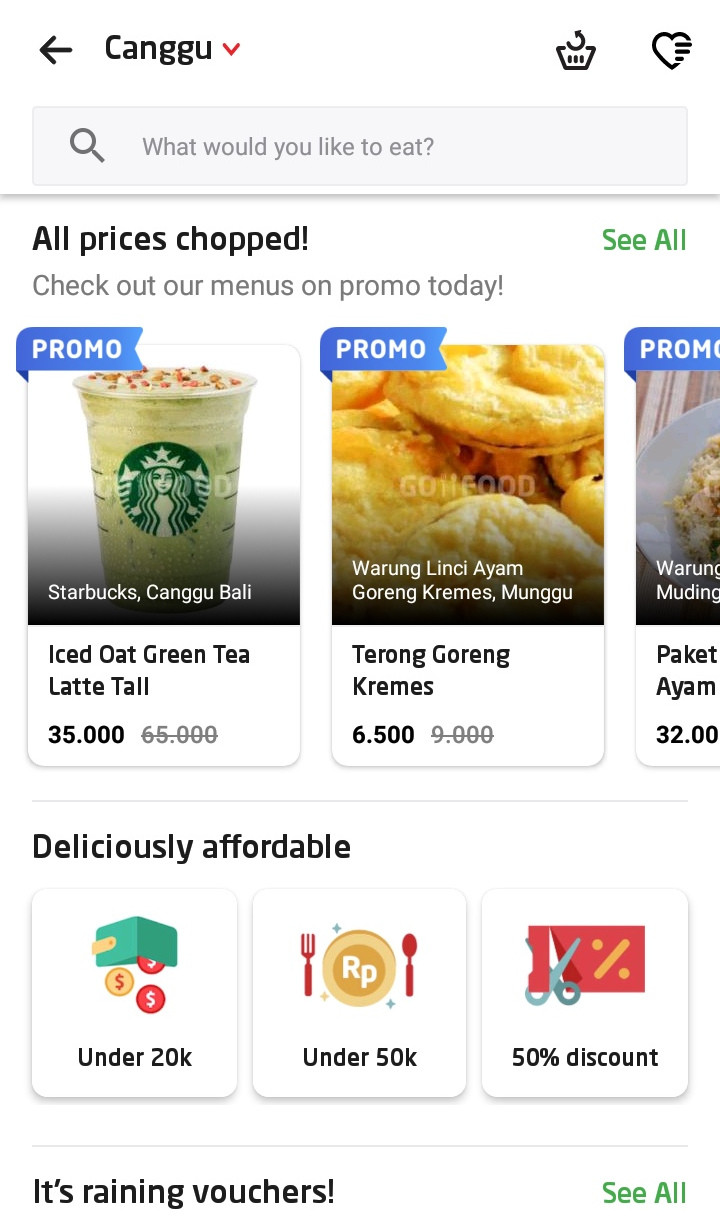The image appears to be a promotional banner for a website showcasing various dining offers. The banner prominently displays the word "CANGGU" in bold black letters, with a left-facing black arrow and a downward-facing red arrow directing attention to different sections. 

The center of the image features a graphic resembling the base of a pot with a half-circle and heart design. Below this graphic is a gray spacebar asking, "What would you like to eat?" and a note that "all prices chopped" with the phrase "See all" highlighted in green.

The promotional information includes:
- "Check out our menus on promo today" with a highlighted section reading "Starbucks Cangu."
- "Iced oat green tea latte," discounted from $65 to $35.
- A banner at the top advertising various promotions, including one for "Tehran Goreng creams" and a partially visible third promo.

Additional promotional details include:
- A statement that reads, "Deliciously affordable under 20K."
- A green box icon with red and gold money imagery.
- A section labeled "Under 50K," illustrating a dish with a red fork and spoon.
- A "50% discount" section featuring scissors cutting a red piece of paper with an orange line and two dots, accompanied by the phrase "It's raining vouchers."
- The phrase "See all" in green.

The visual composition and vibrant colors create an engaging and attractive layout for users seeking food deals and promotions.